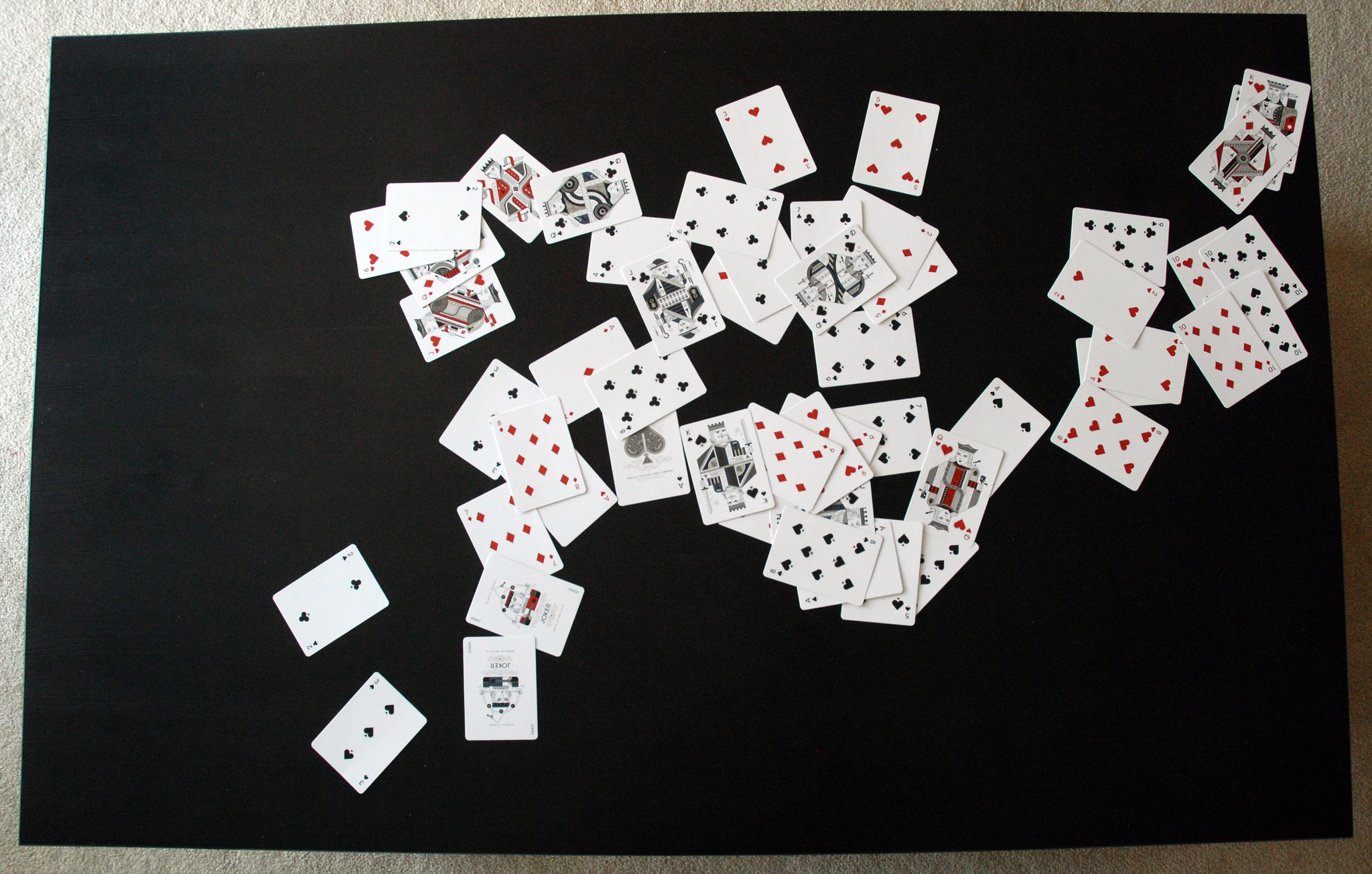This photograph captures a detailed and intriguing composition of a black surface set against a gray, textured wall. The perspective seems to be a downward view, suggesting the black surface lies on the ground, although the interpretation of it being an artwork mounted on the wall remains plausible. Strewn across this black expanse is a full deck of traditional playing cards. The cards, featuring hearts, spades, diamonds, and clubs, along with face cards like kings, queens, and the joker, are artfully arranged. The majority of the cards are concentrated in the center of the black surface, fanning out toward the upper right corner. In contrast, only two cards occupy the lower left corner, while the upper left and lower right corners remain conspicuously empty. The thoughtful dispersion of the cards against the stark black background melds seamlessly with the textured gray wall, creating a visually arresting tableau that blurs the lines between flat surfaces and dimensional art.